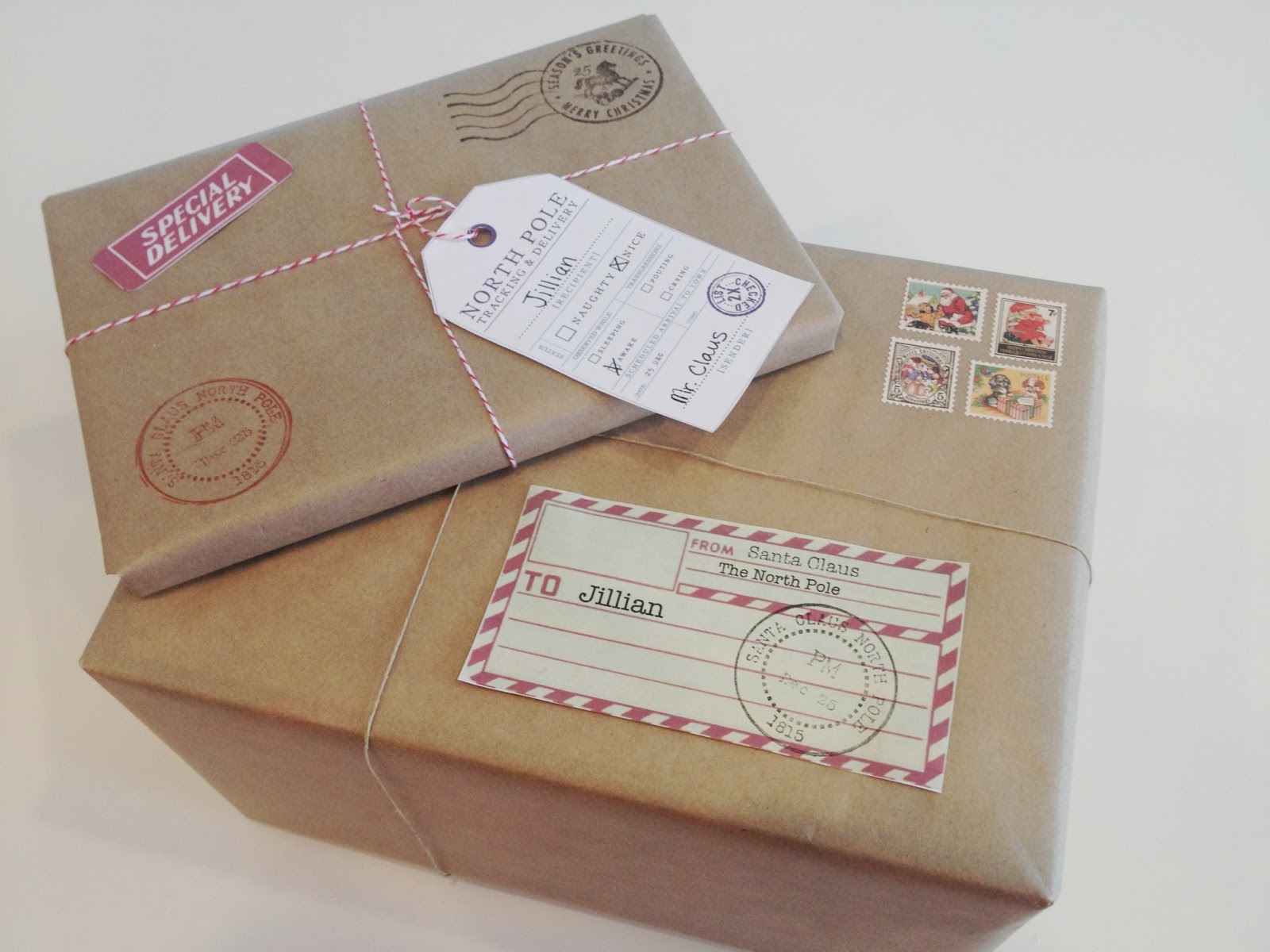This photograph features two packages poised for delivery, set against a light gray background. The bottom package is a large, rectangular box wrapped in brown packing paper. In the upper right-hand corner, it boasts four Christmas-themed stamps arranged in a square. A thin string secures the shipping paper, and a fancy candy cane-striped delivery note on the bottom right reads, "From Santa Claus, the North Pole, to Jillian."

Resting slightly askew on top of this larger package is a thinner, book-sized parcel, also wrapped in brown packing paper. This smaller package is adorned with a pink area in the upper left-hand corner bearing the label "Special Delivery" in white text. It includes a tag that says, "North Pole Tracking Delivery, Recipient: Jillian," with the "Nice" section checked. This is all tied neatly with white and red twine. The sender is listed as "Mr. Claus."